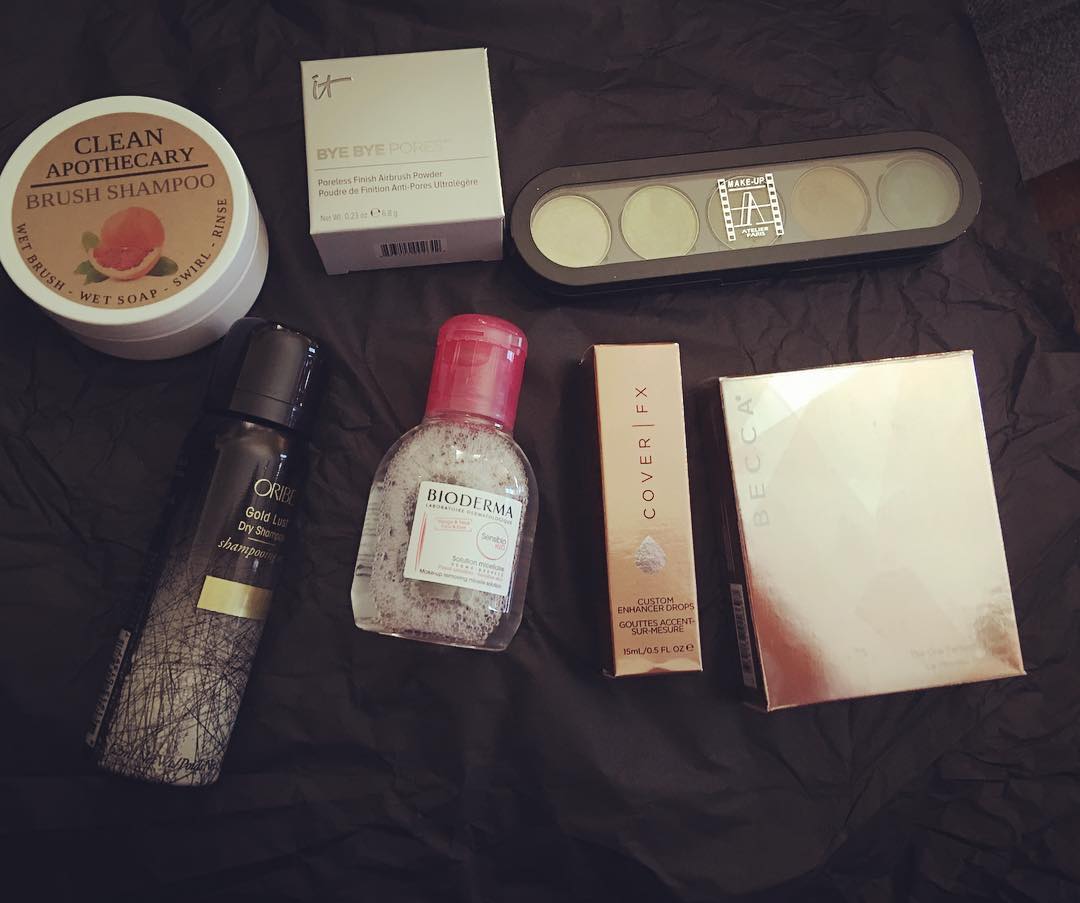An indoor color photograph taken from above showcases a tabletop draped in a black silk cloth, adorned with seven various skin care and beauty care packages meticulously arranged in two rows. 

In the top row from left to right:
1. A small cylindrical jar labeled "Clean Apothecary" with "Brush Shampoo" just below.
2. A square gray box with a label that reads "Bye Bye," partially obscured by glare.
3. A flat, long oval object featuring what appear to be five eyeshadow color samples.

In the bottom row from left to right:
1. A cylindrical bottle with a black cap and a black label fading to gray at the bottom, with "Dry Shampoo" written in gold.
2. A small clear plastic bottle with a red cap, labeled "Bioderma" in black font on a white label.
3. A vertical rectangular gold box marked with vertical text reading "Cover FX."
4. Another rectangular gold box with its print obscured by light glare.

No additional text or details are visible on the packages beyond the descriptions provided.